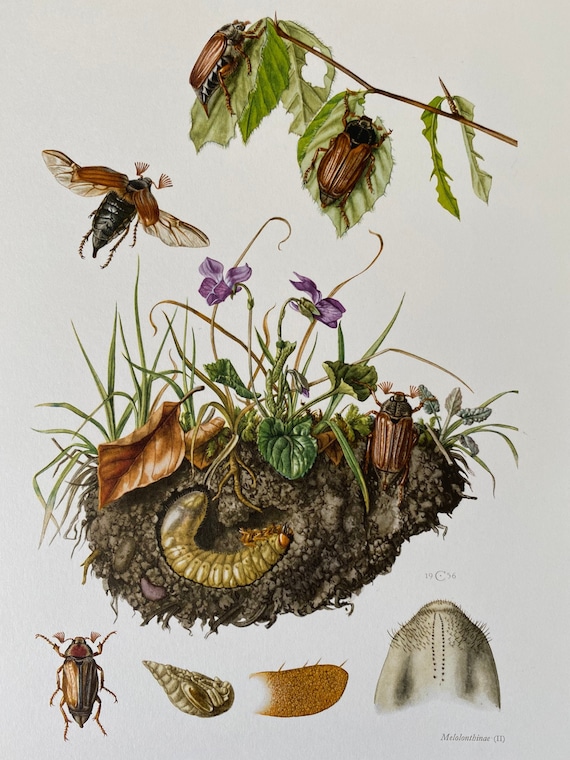This detailed illustration on a white background presents a cross-section view of a dirt field, highlighting various insects and plant life. At the top, a branch extends from the right to the top middle, adorned with several partially-eaten leaves. Perched on two of the top leaves are substantial, brown beetles nearly the size of the leaves themselves. Slightly below, another beetle, similar in appearance, is captured mid-flight with its wings spread. Descending further, the image transitions to a dirt section dotted with small patches of grass and a couple of purple flowers. Within this earthy layer, a green worm can be seen burrowing, and another similar insect is depicted emerging from the ground. The illustration also includes a scattering of seeds, likely to become future plants. At the bottom, the image displays several different insects, with one specifically mirroring the beetles on the leaves above. The other insects, depicted in varying colors and shapes – including one white, another orange, and a tan triangular insect – offer a glimpse into the diverse ecosystem thriving both above and below the soil.